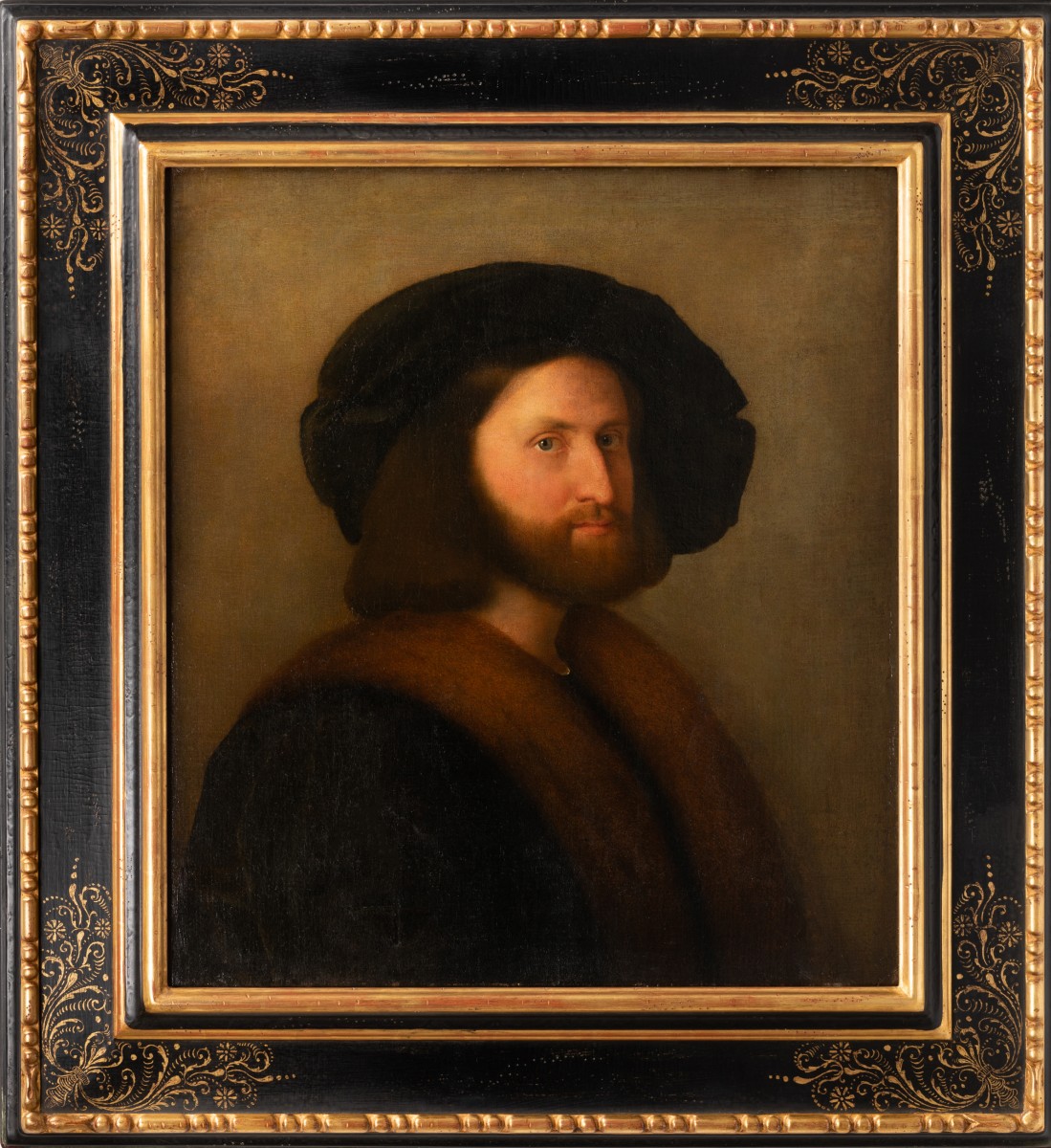A photograph of an elegantly framed painting captures a detailed portrait of a man. The frame is a luxurious black with intricate gold accents at each corner, resembling a crown molding design. Within this sophisticated border, the painting reveals a man with fair skin, brown hair, and a neatly groomed brown beard. He dons a black hat and a black robe or shirt adorned with red accents around the collar and cascading down like a scarf. The background of the painting is a gradient of brown and gray hues, darker around the man's lower section and gradually becoming lighter towards the top, adding depth and focus to the subject's face.